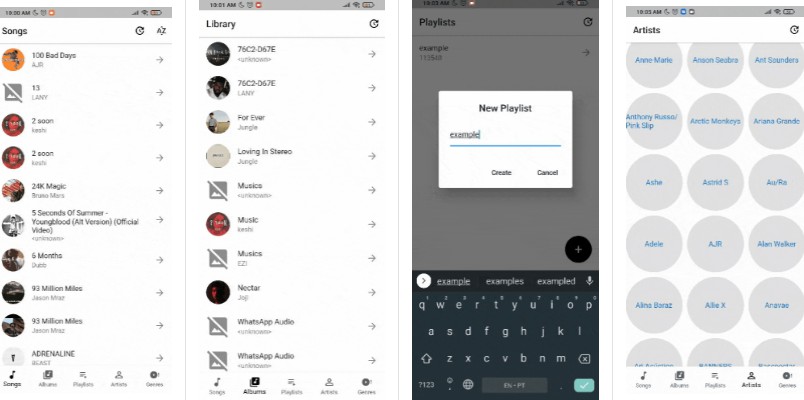A series of four side-by-side mobile device screenshots showcases different sections of a music player application. The first screenshot, on the far left, displays the "Songs" category with a light background. Visible on the left-hand side are small circular icons containing album art, accompanied by the titles of various songs, including Bruno Mars' "24K Magic."

The second screenshot, situated next to the first, is nearly identical but depicts the "Library" section instead. Like the previous one, it features circular album art on the left with corresponding text titles. Some entries, however, lack album art and display a generic gray icon of a snapshot with a strikethrough.

The third screenshot captures a prompt for adding a new playlist. The prompt appears as a white dialog box titled "New Playlist," with the word "Example" typed into the text field.

The final screenshot showcases the "Artists" section, displaying a list of artists in alphabetical order. The left-hand side features circular placeholders where album art would typically appear, but all are blank. The artist names are in blue text, and currently, the letter 'A' is highlighted, with "Adele" being one of the visible names.